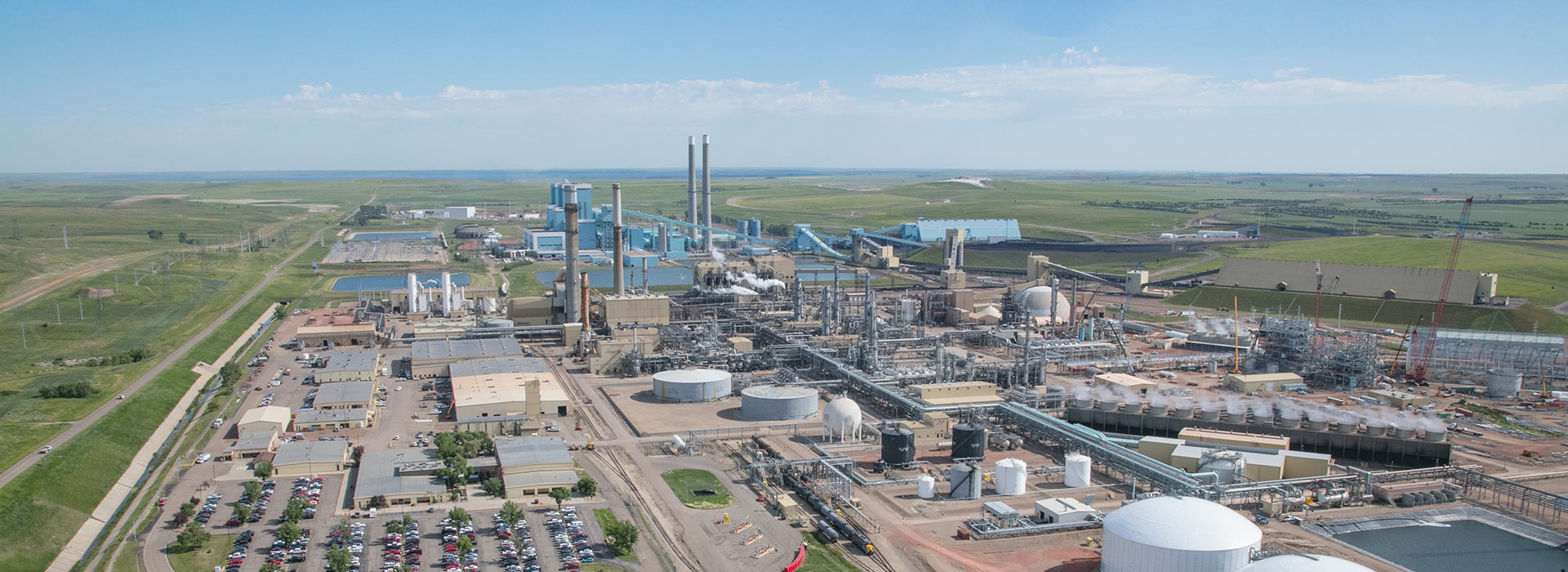This is an aerial photograph of an industrial manufacturing facility, likely a gas or wastewater treatment plant, taken from an elevated location, possibly a drone. The image showcases a sprawling rectangular landscape filled with various industrial components. Centrally located are numerous white storage tanks and smokestacks emitting steam. The facility is threaded with a complex network of pipes and features several gray and sky-blue structures. To the left, a road extends into the distance, while to the right, smaller tanks of a potential refinery can be seen. There are also cranes, including a distinct red ground-based crane on the right, actively moving pipes and aiding in the construction of new facilities. In the lower left-hand corner, there is a parking lot filled with cars, indicating operational activity. Surrounding the plant are open green fields, with no residential homes nearby, only grass, dirt, and roads. Above the industrial sprawl, a light blue sky dotted with clouds completes the backdrop, suggesting the photo was taken in the middle of the day or early evening based on the shadows cast.